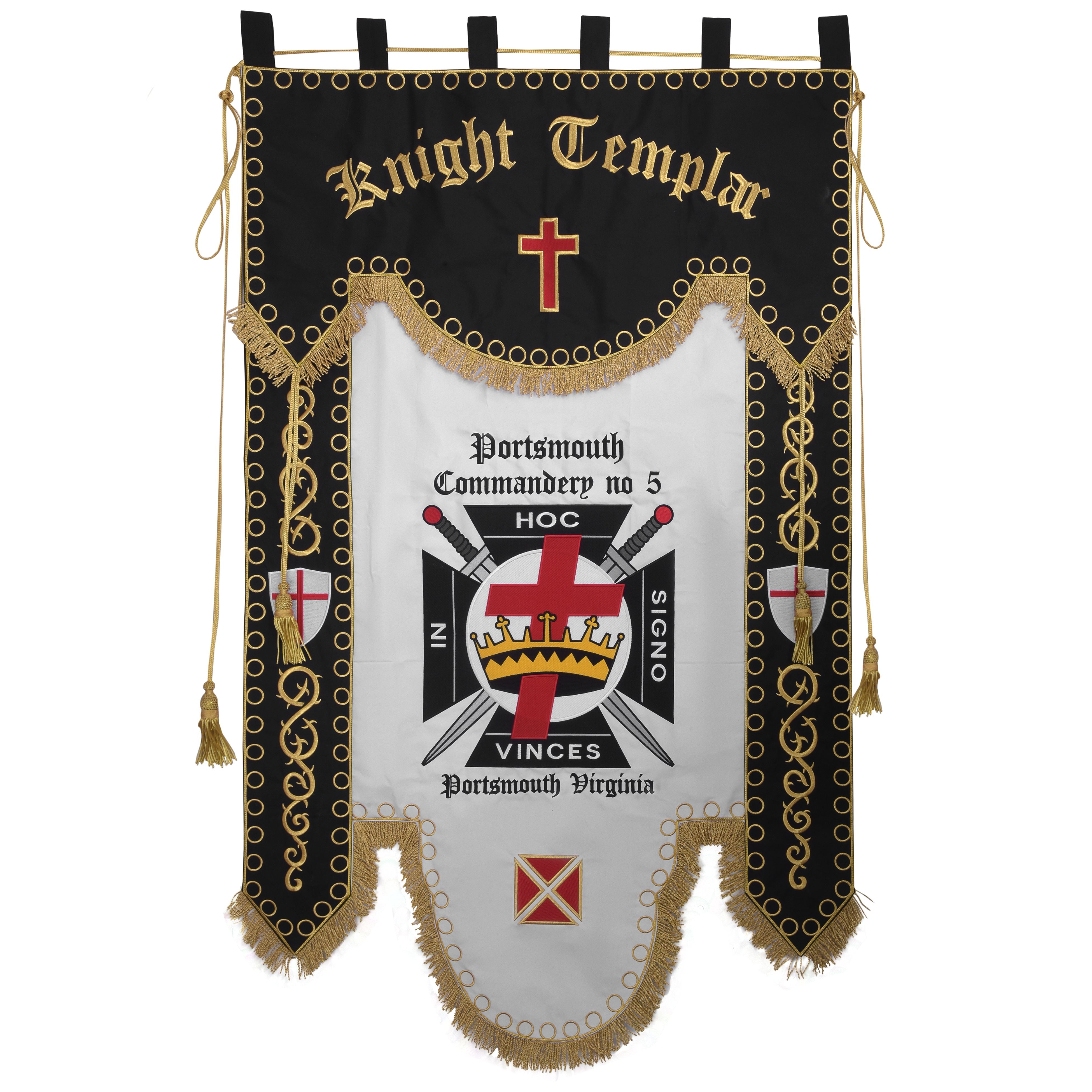The image depicts an ornate banner or standard associated with the Knights Templar, showcasing intricate detailing and symbolic elements. The banner is bordered with golden-colored lining and prominently features a Red Cross. Below the cross, in a white section of the fabric, the words "Portsmouth Commandery No. 5" are inscribed, identifying the chapter. The central emblem includes a crowned Red Cross with two swords crossed diagonally behind it, symbolizing the order. Surrounding the central cross are four key elements: a hawk at the top, a signal to the right, an inn on the left, and fences at the bottom. The banner further specifies its association with Portsmouth, Virginia, highlighting its locality.